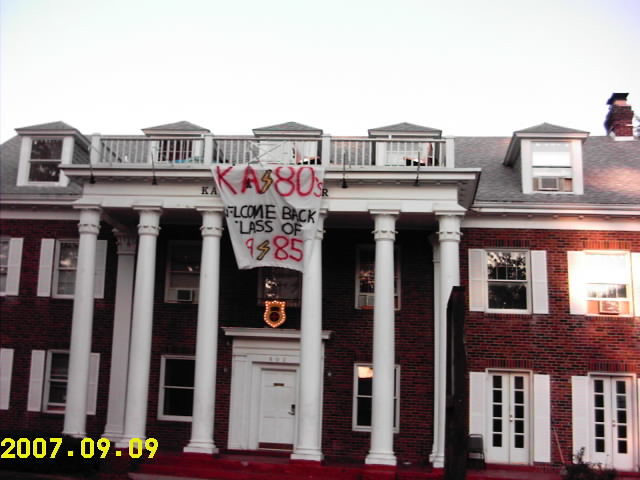The image shows a three-story fraternity house with a red and black brick exterior. The house features six large white columns flanking the white front door, which has a thick white door frame. Above the door is a neon shield-shaped sign, glowing brightly. The lower left corner of the photo displays a yellow date stamp that reads "2007.09.09." The fraternity house has numerous windows; the bottom two floors feature windows with white shutters, while the top floor has windows set into small outcroppings. The building is capped with a gray roof and has a chimney in the upper right corner. A banner drapes across the railing of a balcony that is supported by the columns, stating "KA 80s, Welcome Back Class of 1985," indicating a reunion event. The sky above appears cloudy and bright white.